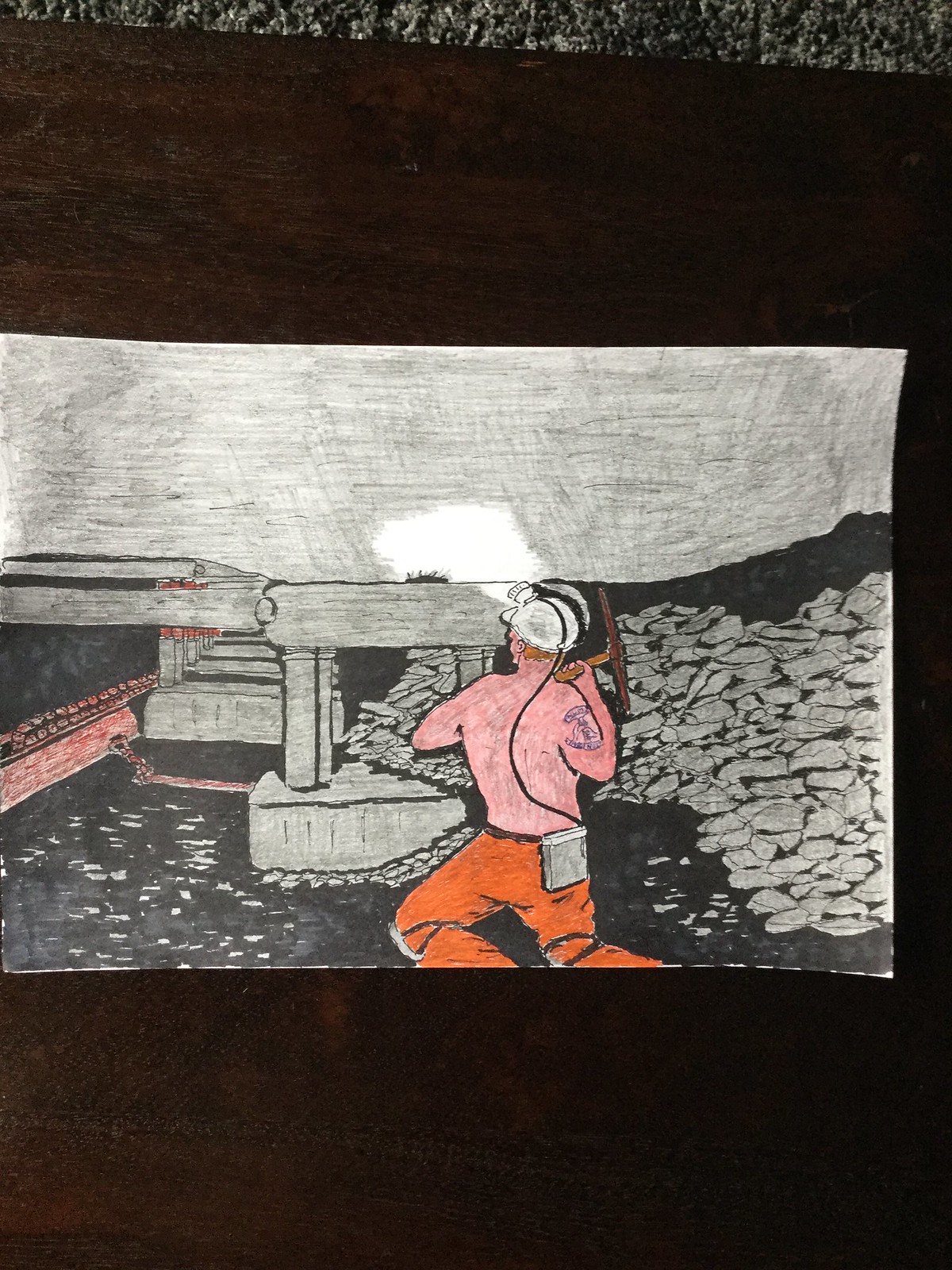The image is a vertically-oriented artwork with a complex, multi-layered composition. The background stands out with three distinct segments. The farthest layer in the back features a textured blend of charcoal and white, set on a diagonal plane which appears to be at the bottom-most level. Dominating the majority of the background is a solid black section. At the forefront lies a prominent piece of art, rectilinear and wider than it is tall, situated towards the left with approximately an inch-wide border visible on the right, thus partially cropping the left side of the artwork.

The central piece appears to be a possibly watercolor, acrylic, or colored pencil work, portraying a rugged miner in fine detail. The miner's bare chest exhibits a pinkish skin tone, accentuated by a bluish tattoo on his right upper arm. He is dressed in white pants, secured with distinctive black straps just below the knees. Notably, the miner wears a helmet equipped with a flood lamp, the associated wire trailing down to a battery pack. The scene convincingly suggests an underground setting with visible rubble scattered predominantly in front of and to the right of the miner, emphasizing the painstaking labor inherent to his environment.